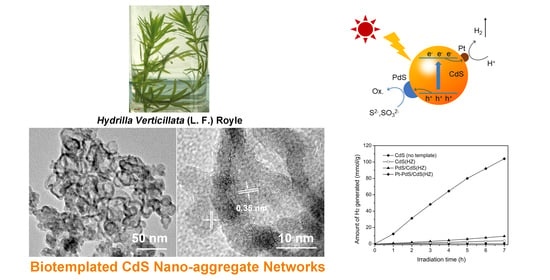The image is an intricate scientific panel on a white background, divided into multiple sections. In the top left corner, there is a label reading "Hydrilla verticulata LF Royal" above a rectangular image of the green plant, resembling a U-shape, with a bluish-gray lower section and an almost beige upper section. Below this, in orange letters, is the caption "Bio-Templated CDS Nano-Aggregate Networks," with two close-up microscopic images labeled 50 nm and 10 nm. One image depicts a vaguely crystalline structure while the other resembles an x-ray with thick black lines and white spots. On the right side, a round orange circle with a blue arrow pointing upward is marked "CDS" or "CAS," accompanied by a red sun icon, a yellow lightning bolt, and various chemical formulas. Below this, a graph with an x and y axis features a line with plotted data points. The collection of images and annotations forms a detailed scientific illustration, likely related to nanomaterial research in biology.